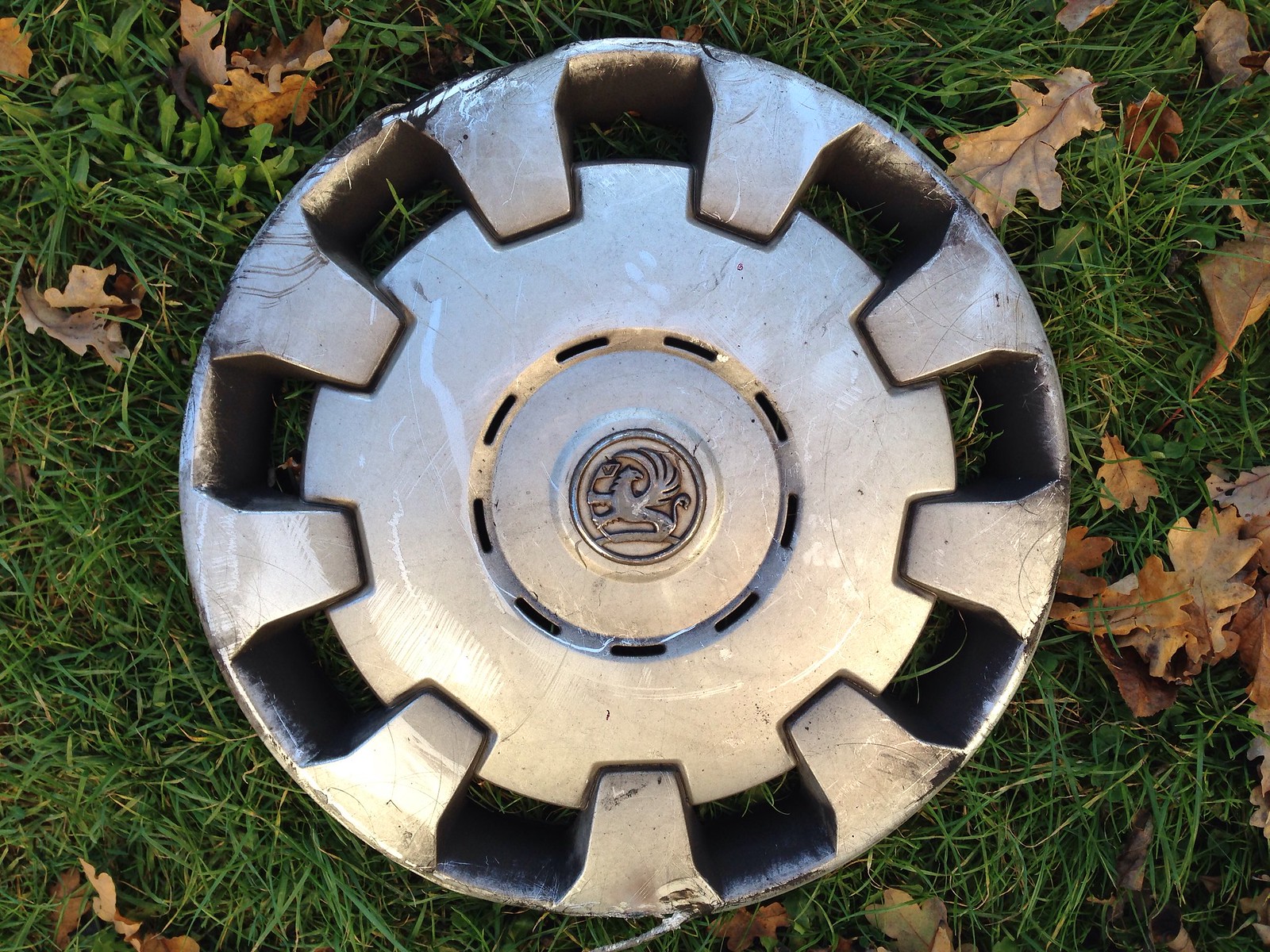The image depicts a top-down view of a hubcap lying on healthy green grass, surrounded by scattered brown and orange leaves. The hubcap is a worn chrome color, with visible tarnish and some bending along its edges. It features a distinctive design with ten dark spoke-like rectangular cutouts connecting to a central metal plate. The centerpiece of the hubcap displays a stylized emblem, possibly a griffin facing right, with intricate details resembling feathers and a lion's tail, suggestive of a high-end car brand. The overall scene captures the hubcap's metallic structure against the natural background, highlighting both the object's ornate craftsmanship and its weathered condition.